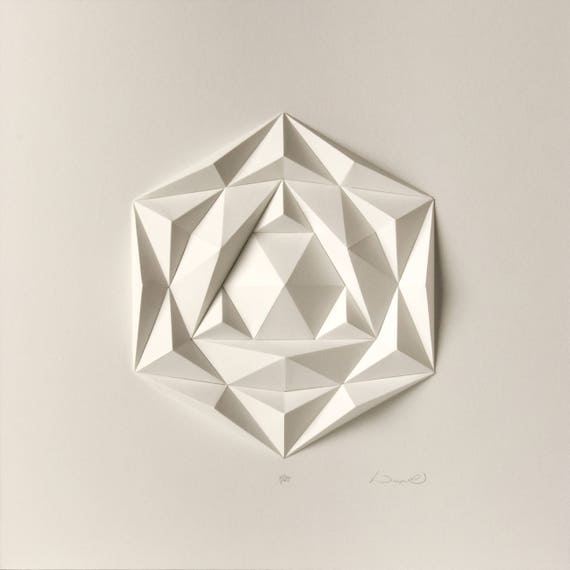The photo captures a meticulously crafted white-on-white geometric art piece with a hexagonal shape, viewed directly from above against a cream-colored background. The central hexagon is intricately layered, resembling the multiple tiers of a wedding cake, and includes various smaller shapes within it, such as triangles, rhombuses, and diamonds, creating a mesmerizing, kaleidoscopic effect. The design evokes the delicate structure of a crystalline flower or a mountainous topography, with folds and crevices adding depth and complexity. Subtle shadows highlight the intricate folds, giving it an origami-like appearance. To the bottom right, there is a faint, barely legible signature from the artist, along with an additional indistinct marking. The absence of strong shadows confirms it was shot directly at its face, emphasizing the detailed craftsmanship of this fascinating piece.